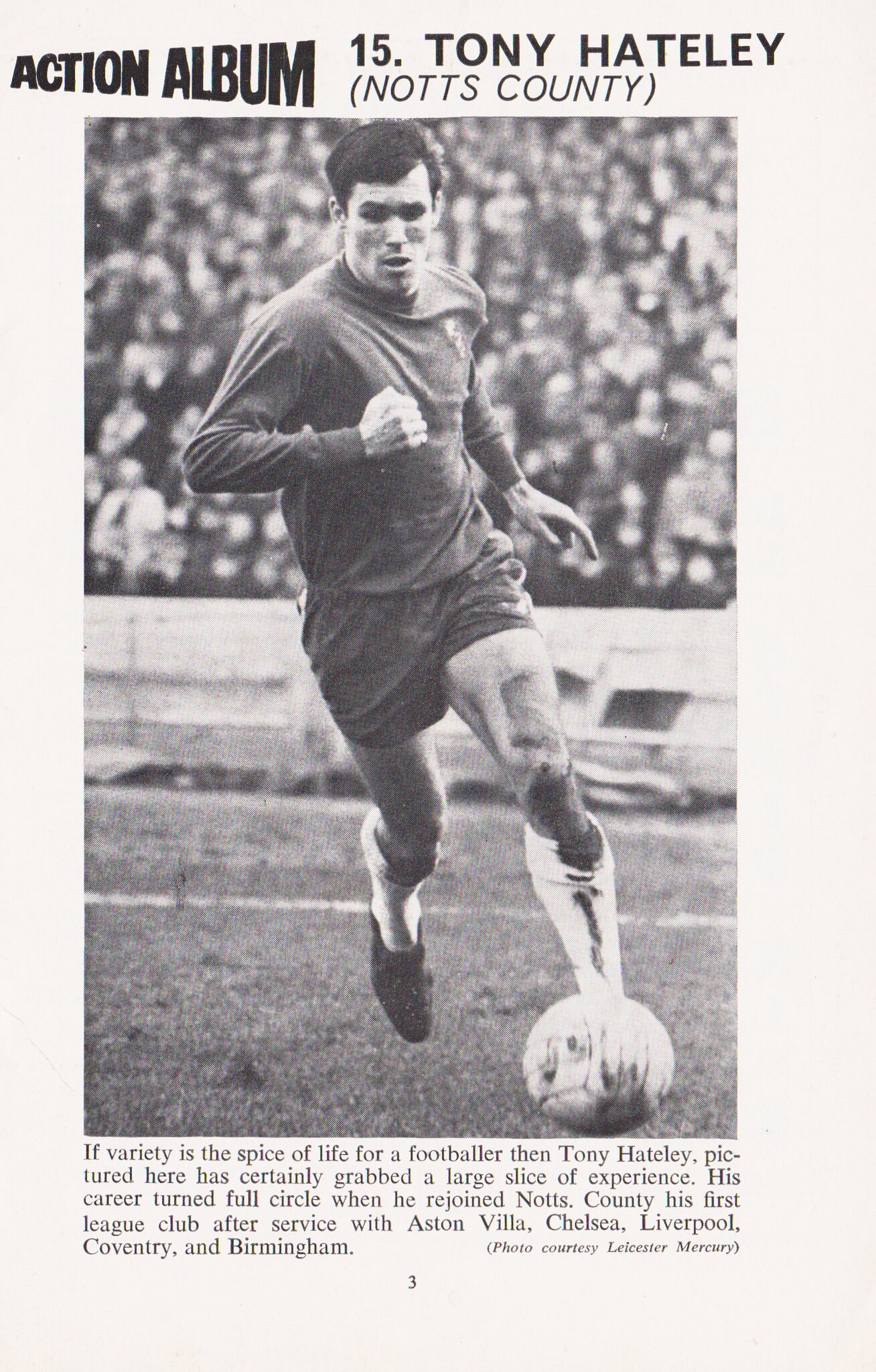The image is a black and white photograph featuring a soccer player identified as Tony Hateley (mislabeled in some versions of the descriptions). The bold header at the top reads "Action Album," with "15. Tony Hateley" adjacent to it, slightly angled to the left, creating an optical illusion of the text moving closer as it progresses. Below Hateley's name is the caption "Notts County" in brackets. The soccer player is dressed in a dark shirt and shorts, with white shin guards and black cleats. He is captured in motion, pushing the ball with his right foot while his left foot is off the ground. His body leans slightly to the left, his mouth open in an oval shape, and he displays a determined expression. His left arm is up, fist clenched beside his bicep, while his right arm hangs loosely behind him. There is text below the image detailing Hateley's career journey, noting that he rejoined Notts County after playing for clubs like Aston Villa, Chelsea, Liverpool, Coventry, and Birmingham. The photo, credited to the Leicester Mercury, shows Hateley against a backdrop of a large crowd, emphasizing his dynamic action on the field. The page number at the bottom of the image is indicated as 3.